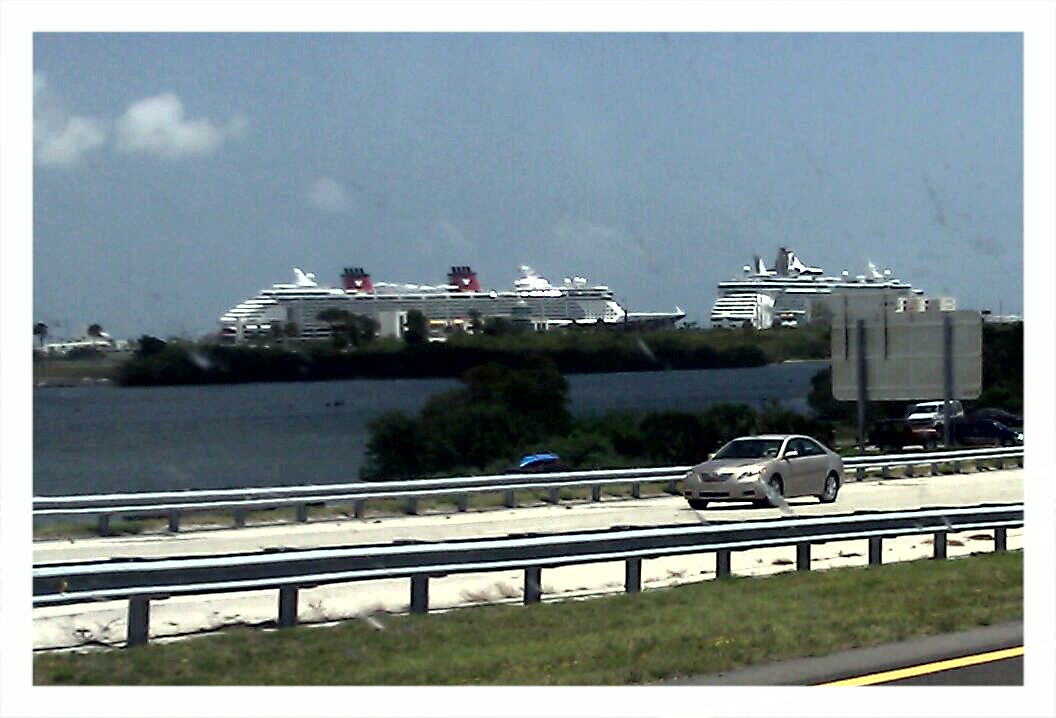The photograph is taken from within a car traveling down a four-lane highway, capturing a detailed scene likely set in Florida. In the foreground, a light gold or silver car drives on the left side of the highway, while the observer's car moves in the opposite direction on the right side, partially obscured by some dirt on the window. On the right of the image, a grass median separates the lanes. The highway runs adjacent to an inland waterway, framed by trees and shrubs that grow right up to the water's edge. Beyond the two lanes of the highway and across the waterway sits a row of enormous cruise ships, reminiscent of the ones used by Disney—identifiable by red smokestacks topped with blue and featuring the iconic Mickey Mouse insignia. One of the ships' superstructures, painted white with areas designated for passenger accommodations, stands prominently against the horizon. This scenic backdrop includes a large body of water and possibly an island, enhancing the tranquil yet bustling environment.